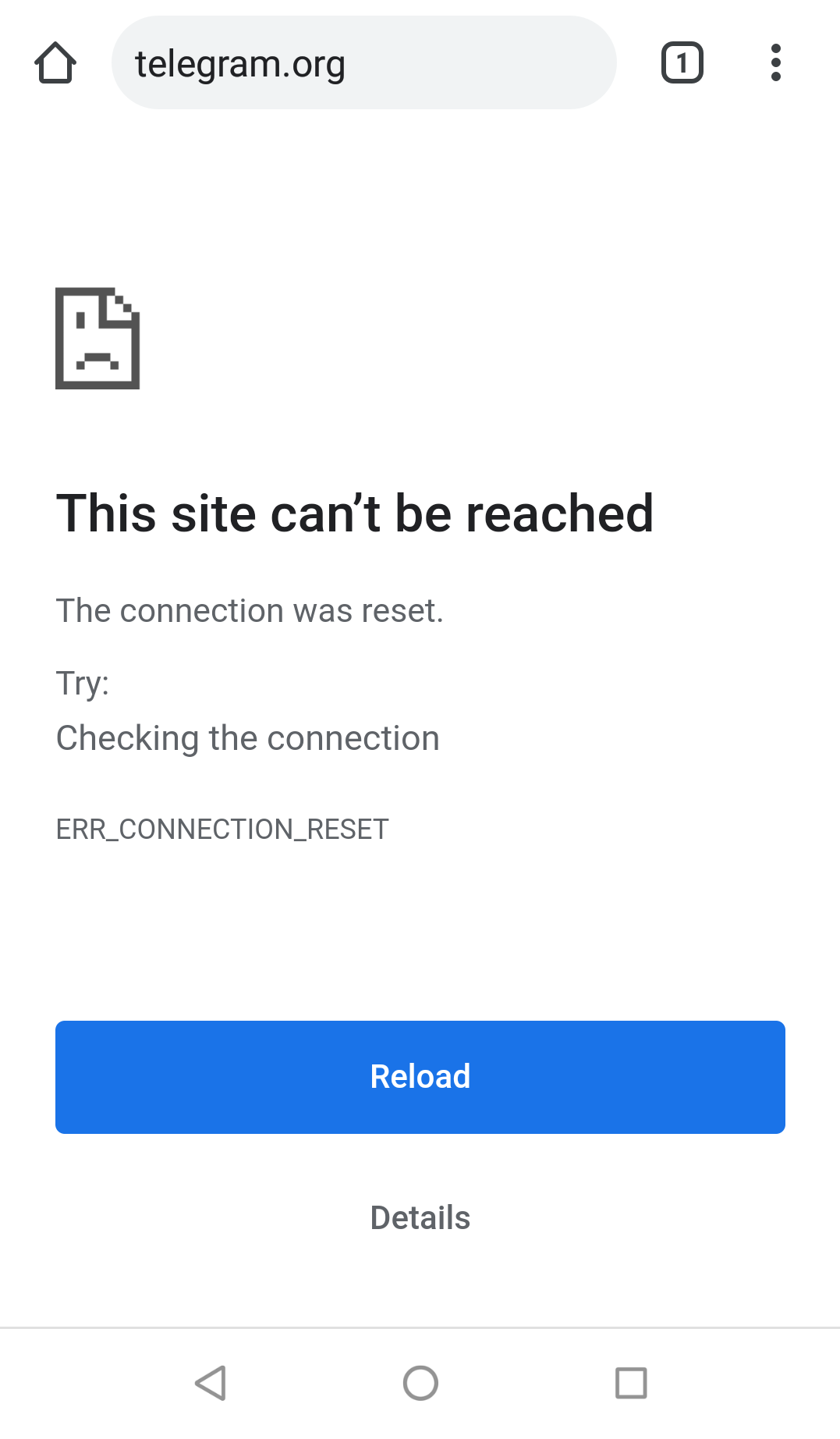This image is a screenshot from a phone displaying an error message on a web browser. The background is predominantly white. In the top left corner, there's an icon of a stick house. Adjacent to it, there is an oval shape with a gray background containing the text "TELEGRAM.ORG." Below this, there is a small square with the number "1" inside it, followed by an ellipsis (three dots). 

Further down, there is a section with white space featuring an image of a cartoon-like piece of paper with a bent top right corner. The paper shows a single eye and a sad mouth, symbolizing an error. Underneath this illustration, bold black text states, "This site can't be reached." Below this message, regular black text reads, "The connection was reset."

Following this, there are instructions starting with "Try..." and the first suggestion is "Checking the connection." Under these suggestions, the text "ERR_CONNECTION_RESET" is displayed in all caps with underscores.

Towards the bottom of the screen, there is a wide blue button with the word "Reload" and a "Details" option next to it. Below these options, a thin gray line separates the content, leading to icons of a triangle, a circle, and a square at the very bottom.